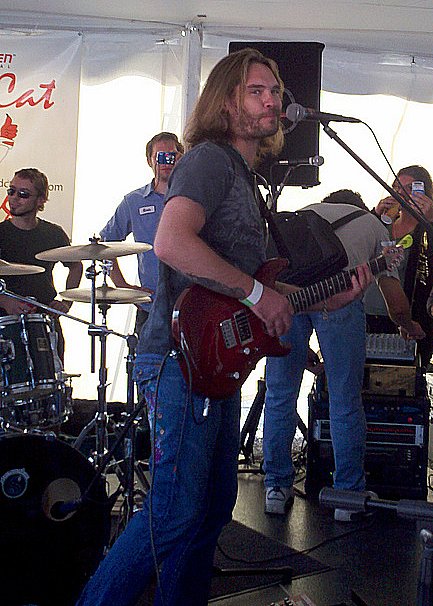The image features a dynamic scene of a band preparing for a concert under a covered tent. Central to the image is a long-haired musician with a slight beard and mustache, wearing blue jeans, a gray t-shirt, and a white wristband. He cradles a red electric guitar and stands in front of a microphone, looking to his right with a smug, almost smiling expression. His right arm displays a tattoo. 

In the background, a drummer with sunglasses is positioned behind a full drum set. Part of a poster with red letters on a white background is visible behind him. To the left of the drummer and over the guitarist's right shoulder, a man in a blue shirt, potentially with a name label, is seen wearing sunglasses. 

On the right side of the image, a man is adjusting a tall speaker, while a woman behind him is sipping a cup of coffee. Additionally, another person dressed in black is visible in the audience, and a blue-shirted individual appears to be taking a picture. A tent pole can be seen in the center, contributing to the sheltered setup of the scene.